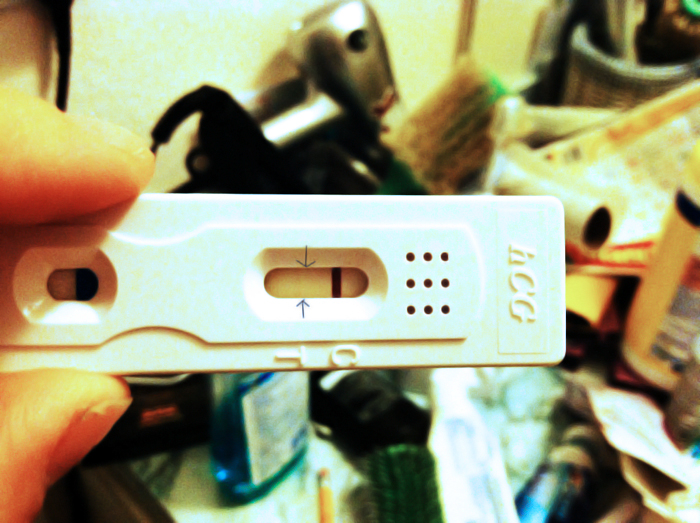In this image, an individual is holding a home-use pregnancy test horizontally between their thumb and index finger. The beige HCG test displays one prominent dark line and a very faint second line, almost imperceptible, marked by two arrows on the indicator. The sample area of the test is clearly visible. The background reveals a cluttered room with nearly empty paper rolls, tissue dispensers, and what appears to be a mouthwash bottle beneath the test. Among the scattered items are a pencil, suggesting the scene is atop a desk. The far wall in the blurry background is an off-white color, contributing to the overall disorganized appearance.